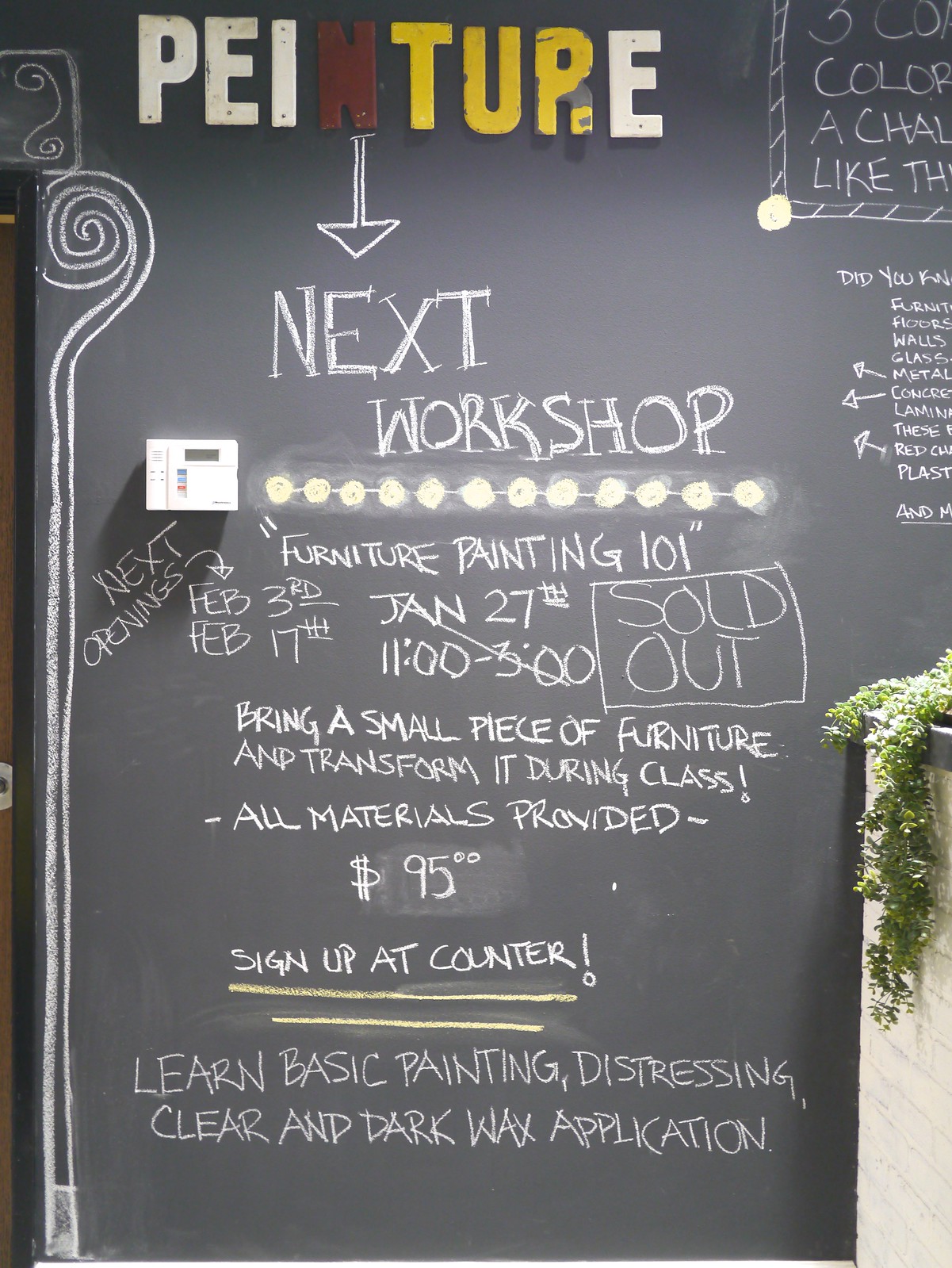The image is a detailed chalkboard advertisement set against a black background. At the top center, the word "PEINTUP.E" is prominently displayed with distinctive coloration: "PEI" is white, "N" is red, "TUP." is yellow, and "E" is white. Below this, a white chalk arrow descends from the "N," directing attention to the text "Next Workshop." Scattered around this are small circles and dashes, resembling decorative lights. 

Beneath this section, the board lists "Next Openings" alongside "Furniture Painting 101." The dates "February 3rd," "February 17th," and “January 27th” (crossed out and marked "Sold Out") are provided, indicating the workshop schedule from 11 AM to 3 PM. 

Additional details include: "Bring a small piece of furniture and transform it during class. All materials provided. $95. Sign up at counter!" which is underlined twice for emphasis. Lastly, the bottom of the board reads: "Learn basic painting, distressing, clear, and dark wax application," outlining the workshop’s curriculum.

The setting is captured clearly and brightly, suggesting the image was taken in a well-lit environment. The left side of the board includes a small device with a screen. The top right corner of the board features additional text, partially visible but cut off from the full view.